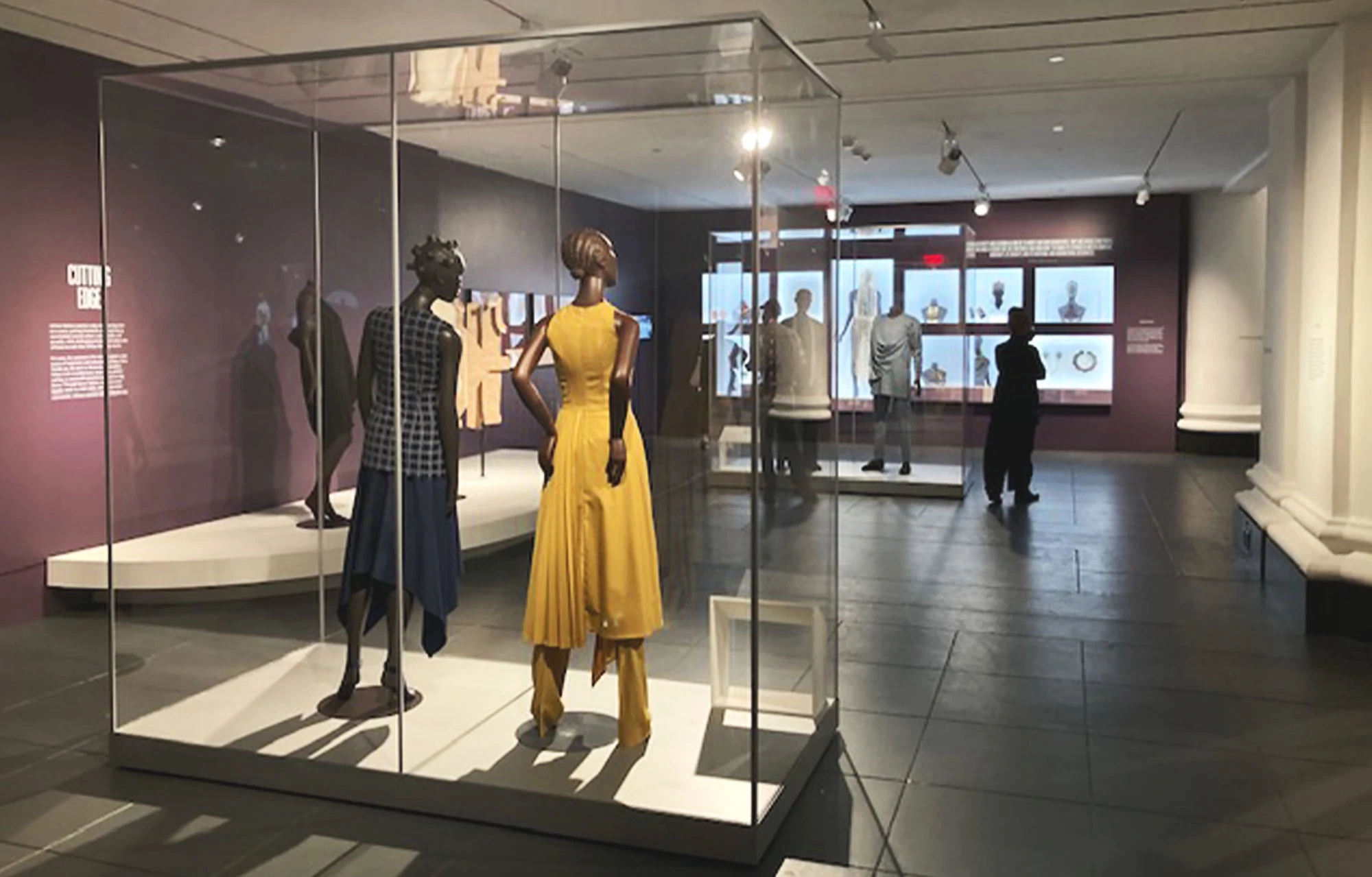The photograph depicts a highly curated exhibition space reminiscent of a museum, possibly a fashion gallery or a high-end designer studio. The room is expansive and modern, with several glass display cases housing full-body mannequins adorned in elegant dresses and pantsuits. One prominently featured mannequin is dressed in an eye-catching yellow outfit, while another wears a blue dress. The layout suggests a museum ambiance, accentuated by dim lighting and strategically placed spotlights that highlight the displays, creating an atmosphere of refined aesthetic appreciation. Text on a dark wall in the background hints at further context, though it remains unreadable. Amidst the mannequins, which include both head and bodice forms displayed in glass cases, stands a lone figure, possibly a visitor, adding to the sense that this is a space meant to be viewed and admired. The overall impression is one of sophistication, suggestive of either a museum exhibition or an extraordinarily luxurious retail experience.